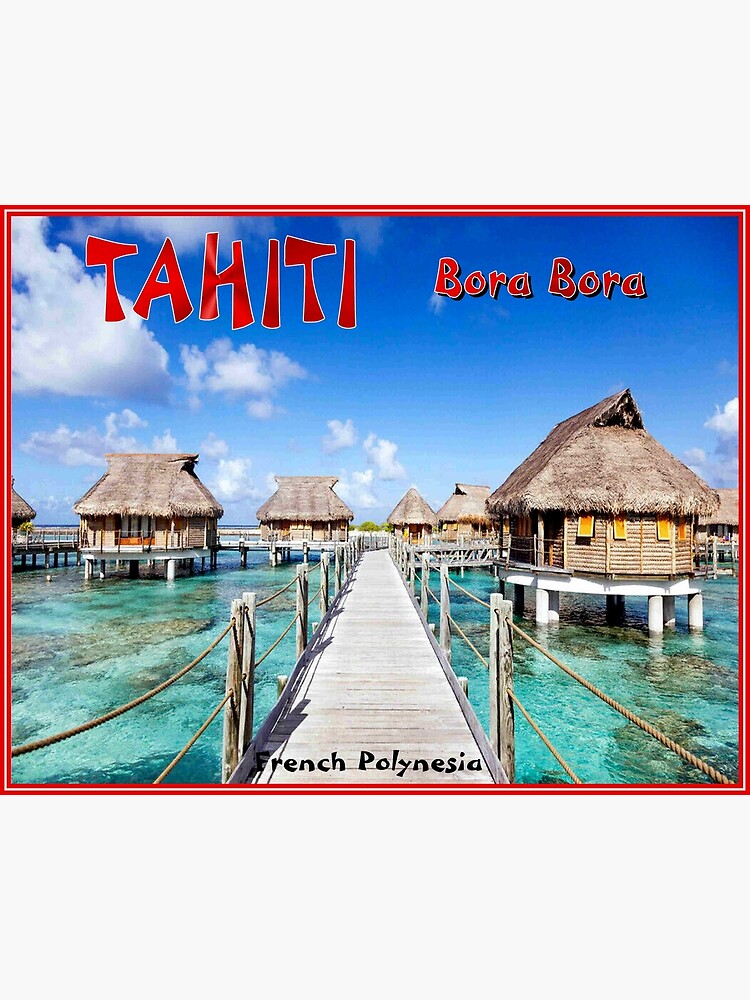This image has the appearance of a postcard, complete with a red border around the edges. At the top, in a stylized Polynesian font, it says "Tahiti" in all caps in the upper left corner, and "Bora Bora" with regular capitalization in the upper right. At the bottom center, written in smaller black font is "French Polynesia." The photograph captures a picturesque resort scene with several huts perched over a mesmerizing teal-blue water, where the seabed's rocks are visible through the clear water. The huts, characterized by their straw or grass roofs, are supported by wooden stakes that elevate them above the water's serene surface. Above the horizon, the blue sky is almost cloudless, adding to the idyllic atmosphere. A wooden boardwalk or bridge with rope railings runs down the center of the image, inviting viewers to imagine strolling between the charming over-water huts in this tropical paradise.